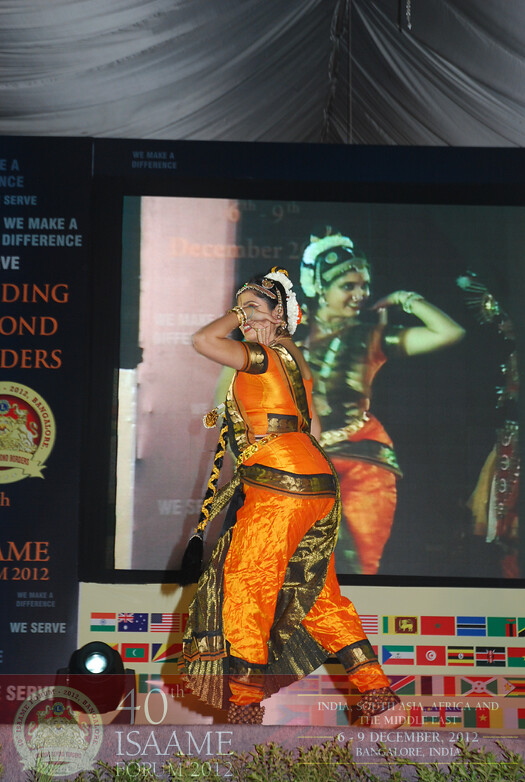The photograph captures an Indian woman standing on an indoor stage, possibly performing or dancing, dressed in a vibrant and festive orange outfit with gold accents. The attire includes long braids wrapped with orange rope and a distinctive headdress with white feathers, somewhat resembling a crown. She is adorned with numerous pieces of jewelry on her wrists. The background features a large screen displaying her from a frontal perspective, whereas the main image shows her from the left side. Her left hand is raised to her cheek while her right hand is out of sight. A black curtain or tent drapes overhead, and below the screen is a white horizontal poster adorned with the flags of various countries. Text at the bottom of the image reads: "40th Esame Forum 2012, India, South Asia, Africa, and Middle East, 6-9 December 2012, Bangalore, India." Additionally, a sign with colored words and the phrase "We Serve" is visible.